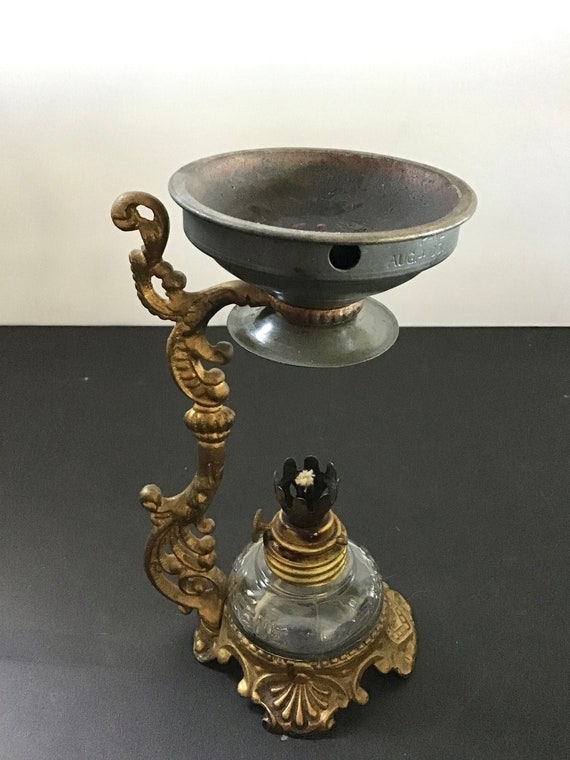This photograph captures an intricate Victorian-style lamp, likely an antique artifact that might be showcased in a museum. The lamp is positioned on a dark surface against a white wall, and the image is taken from a slight angle. The lamp features a brass and glass base, designed to hold kerosene. At the top, a wick is encased in a black holder, with a knob on the left to adjust the wick's height. Above the wick, a small, weathered steel bowl is held by an elegant, pillar-like brass neck. This bowl could possibly be used for heating substances like medicine. The craftsmanship and materials—brass, glass, and metal—highlight the intricate and elaborate design characteristic of the Victorian era.